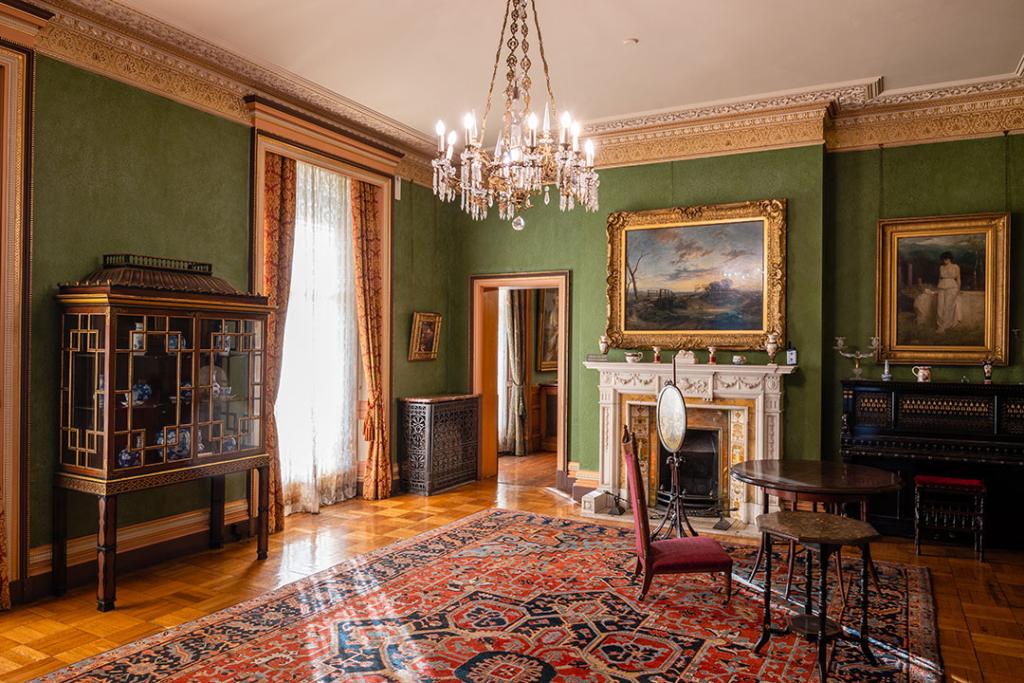The photograph captures an exquisite Victorian-style interior, likely of an antique mansion or a finely decorated home. The room features green walls adorned with intricate crown molding and gold accents that transition into an off-white trim. The highly polished, checkered wooden floor showcases a large, red, white, and blue Persian rug with floral patterns. 

At the room's center stands an ornate white fireplace with elaborate gold filigree. Above it hangs a framed painting, complemented by another framed artwork to its right. A grand chandelier with candle-like lights illuminates the space from above. 

To the left, windows stretch from floor to ceiling, draped with heavy, luxurious curtains. A glass bookcase filled with blue and white china adds to the room's opulence. A piano or organ with a dark brown lacquered finish and red velvet seat is situated near the right wall, along with a low red velvet chair, a small coffee table, and a multi-legged mirror.

Additional elements include a hutch with brass detailing, adding to the overall Victorian charm, and a doorway leading to another richly decorated room in the background.